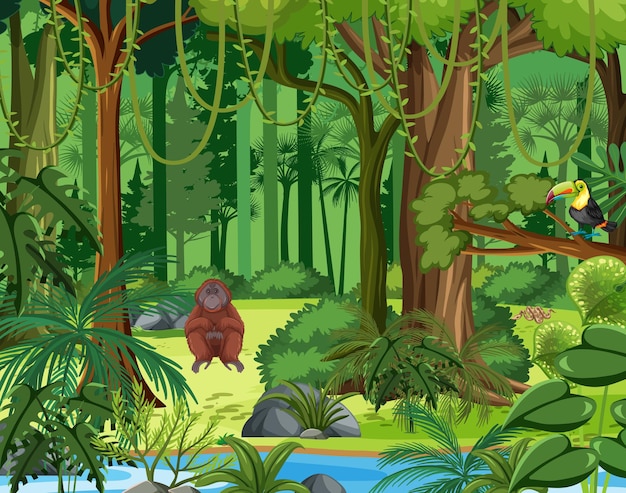This detailed cartoon artwork illustrates a vibrant jungle scene centered around an orangutan with reddish-brown fur sitting on the ground. A blue river, bordered by a mound of land, flows across the bottom of the image, with tufts of green foliage sprouting from rocks in the foreground. The scene displays an abundance of varying trees with brown trunks and green hanging vines cascading in U-shaped curves from the top. To the center right, a toucan with a strikingly colorful beak—displaying shades of green, purple, and blue—and a yellow face, perches on a branch, gazing towards the orangutan. The overall atmosphere is one of lively, dense jungle life, making the illustration highly detailed yet simple in its vector art style.